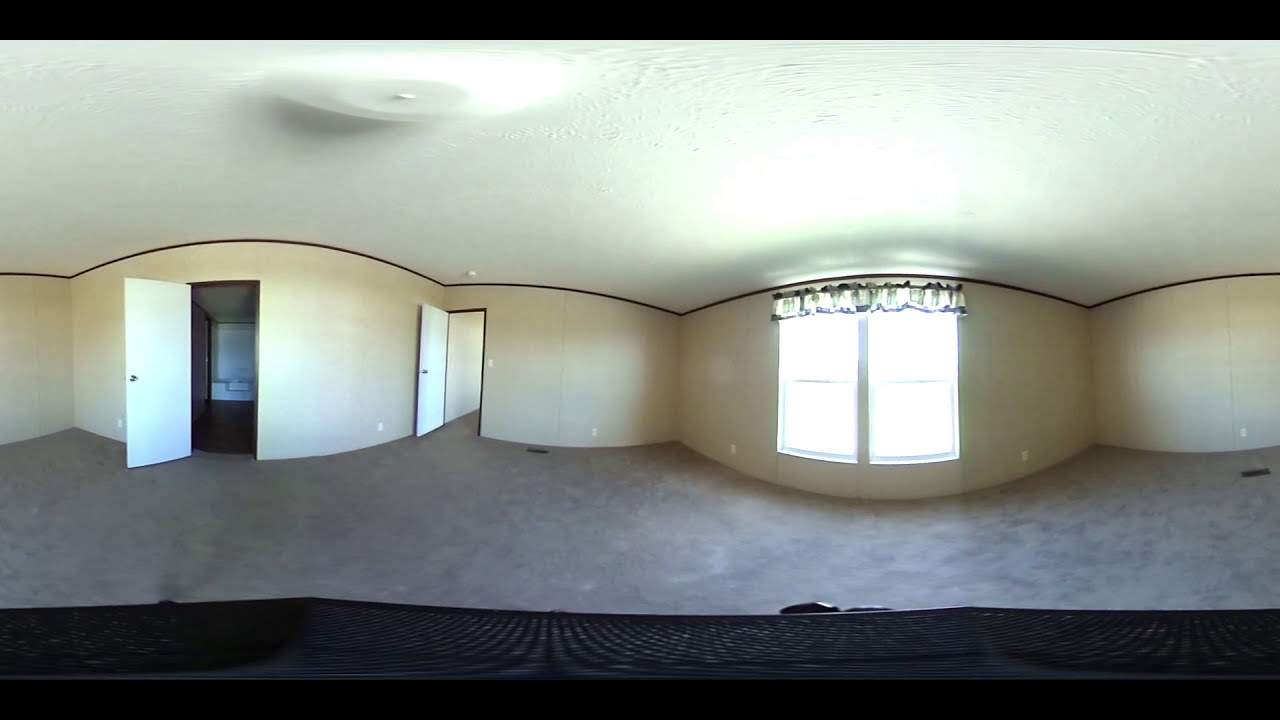The image depicts a spacious, panoramic room with light beige walls and off-white, arched ceilings, creating a distinct segmented effect. The ceiling is white, while the floor is covered in a gray-beige carpet. The room features two doors: one appears to lead to a closet, with a brown floor visible inside, and the other opens to a hallway with the same carpeting extending out. A pair of double windows, adorned with a patterned valance, are situated on one wall, letting in ample sunlight that casts a glare on the room and wall shadows. There's a dark, net-like area at the bottom of the image, and some sort of vent is located on the floor. The room is also noteworthy for an unusual bulge descending from the ceiling.